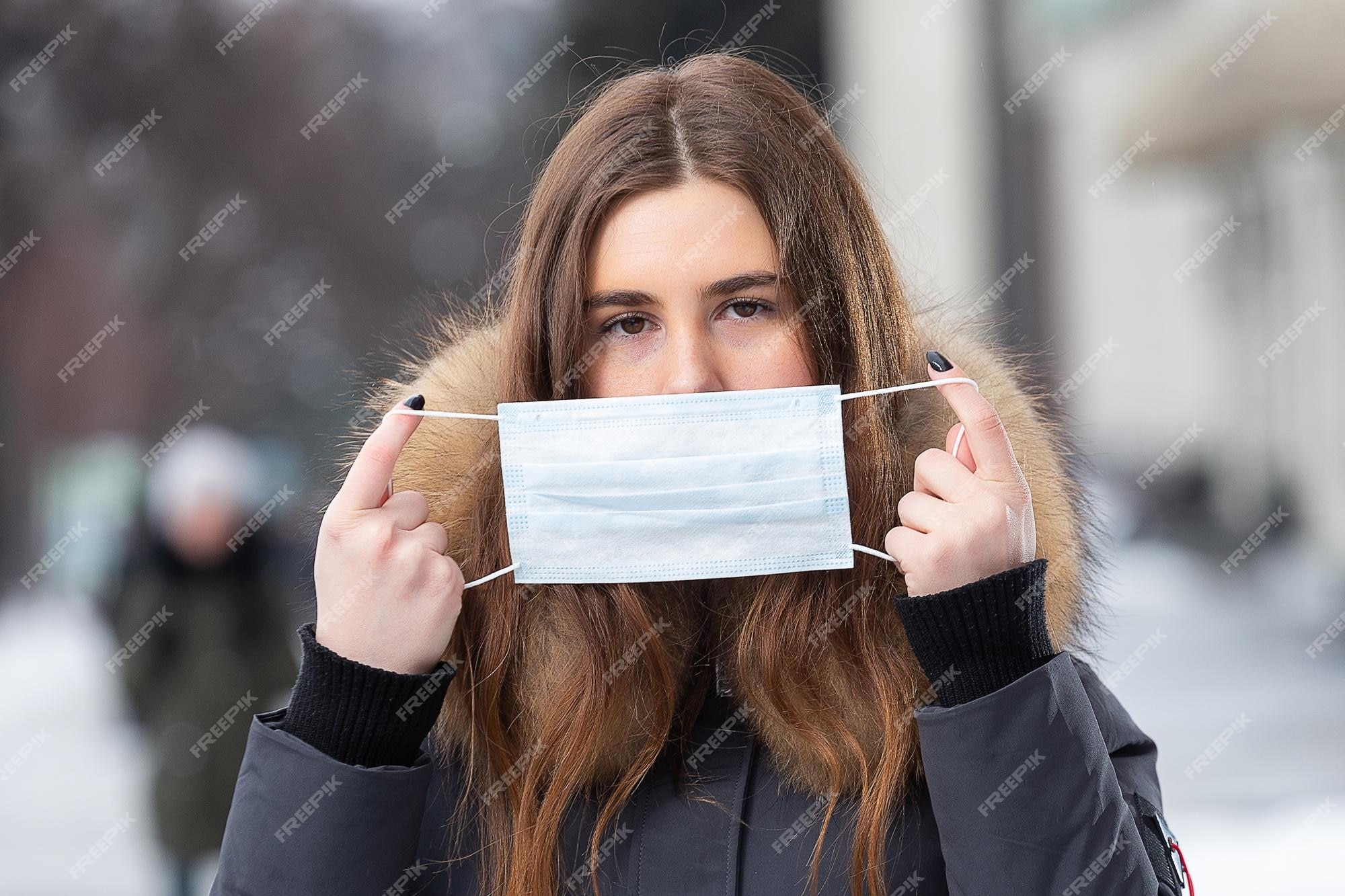In this color photograph, a young Caucasian woman in her 20s with light skin and long auburn brown hair stands outdoors, wearing a gray winter coat with a furry brown and beige collar and black wrist cuffs. Her black fingernails are painted, and she holds a light blue disposable surgical mask stretched out in front of her face, partially covering her nose but not her eyes, revealing her brown eyes which have a neutral expression. The background is blurred, showing indistinct people walking and buildings. There is a noticeable watermark that says "Freepik" running diagonally across the image.